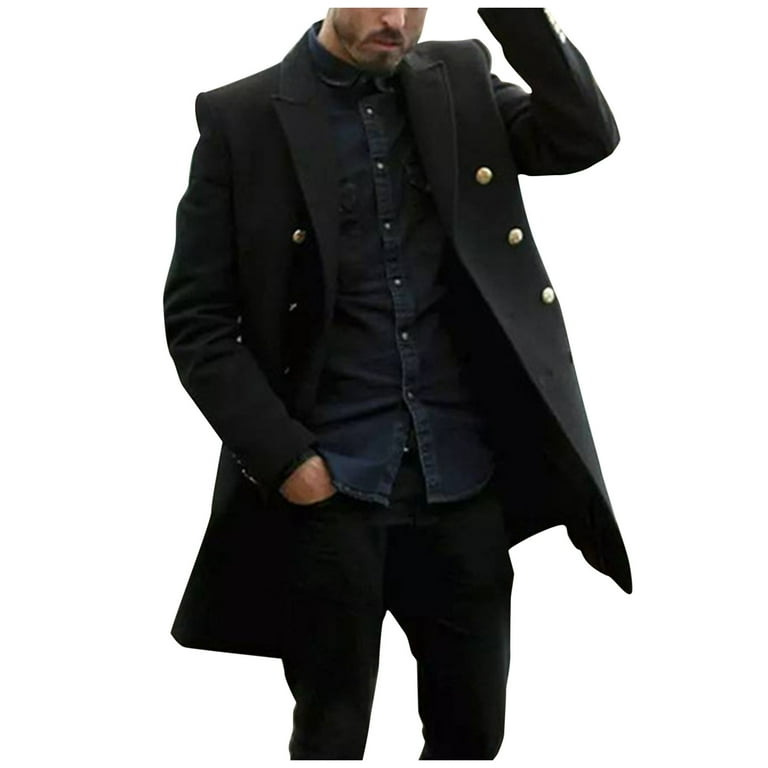In this photograph of a man against a stark white background, the subject is modeled in a sophisticated and slightly eclectic ensemble. The man, who has a short-shaven beard and goatee, is dressed in a striking black overcoat that extends to just above his knees. This coat features padded, triangular shoulders and six prominent, gold-colored round buttons, three on each side, which embellish the breast area. Beneath the overcoat, he wears a dark blue, button-up denim shirt with a collar, tightly fastened except for the last button at the bottom. His trousers are black jeans, complementing the overall dark palette. The image is cropped from the man's nose down to his knees, with his right hand casually tucked into his jeans pocket while his left hand rests by his head, possibly touching his hair. The tight sleeves of the overcoat and the precision of his attire, combined with the white background, give the image a distinct modeling vibe.